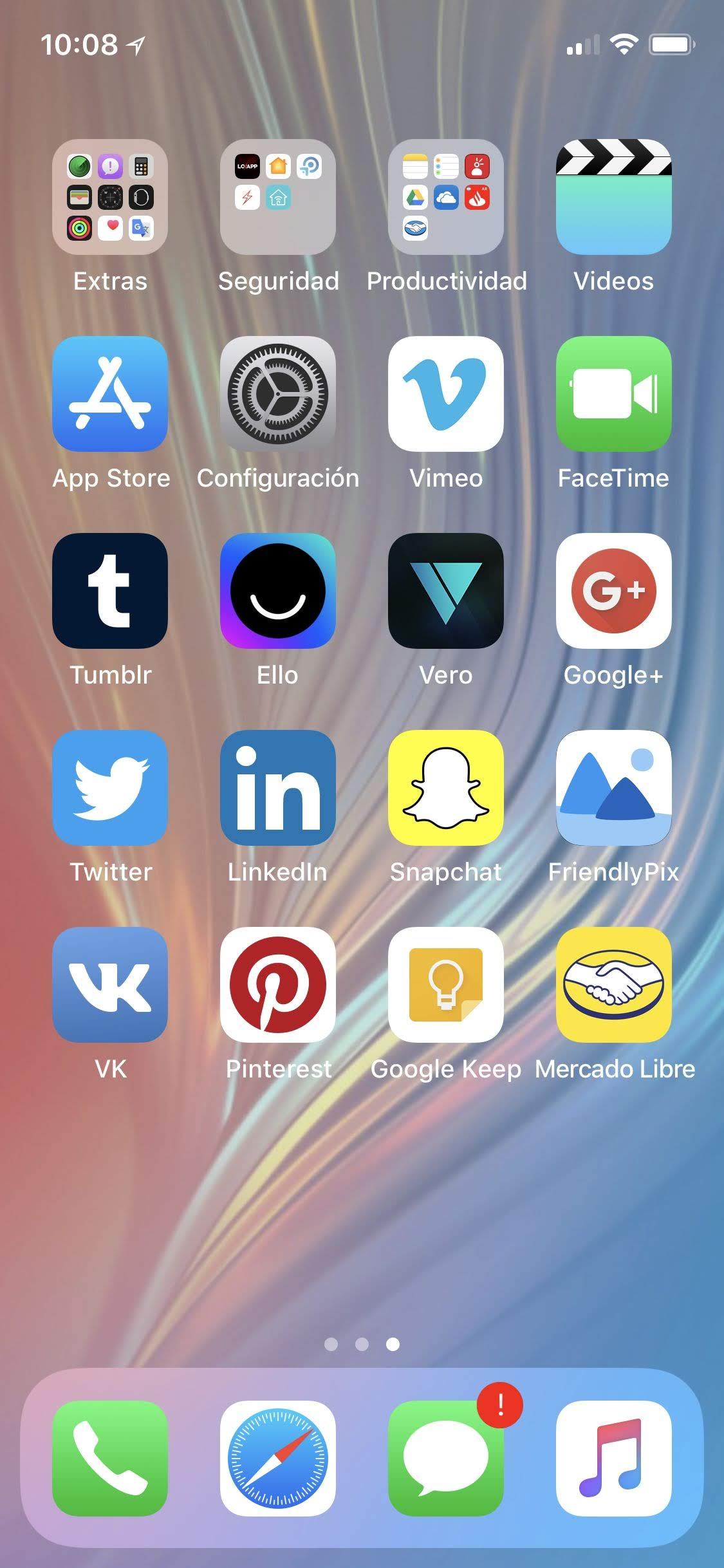The image is a detailed screenshot of a smartphone's home screen. The background of the screen features a light-toned swirl of colorful lines, resembling either high-speed headlights or elegant curves. In the top-left corner, the time is displayed as 10:08 with a northeast-facing directional arrow. On the top right, there are several icons: a weak signal bar, a WiFi symbol, and a fully charged battery icon.

The home screen contains five rows of app icons. At the bottom of the screen, there are standard icons for the phone's core functions: Phone, Compass, Messaging (featuring a red circle with an exclamation point indicating a push notification), and Music.

The app rows are organized as follows:

1. **First Row:** 
   - Extras (organized into a folder)
   - Seguridad (Security settings)
   - Productividad (Productivity apps)
   - Videos (featuring a clapperboard icon styled against a blue background)

2. **Second Row:**
   - App Store (marked with an A)
   - Configuración (Settings, depicted with a set of gears)
   - Vimeo (blue background with the Vimeo V logo)
   - FaceTime (green square with a white video camera icon)

3. **Third Row:**
   - Tumblr (black square with a lowercase T)
   - Ello (blue and purple square with a black smiley face, no eyes, just a white smile)
   - Vero (black background with a stylized V logo)
   - Google+ (white square with a red circle and a G+ symbol)

4. **Fourth Row:**
   - Twitter (blue square with a white bird logo)
   - LinkedIn (blue square with white IN letters)
   - Snapchat (yellow square with a white ghost)
   - Friendly Pix (white background featuring blue mountains, a blue ground, and a blue sun)

5. **Fifth Row:**
   - VK (blue background with conjoined V and K)
   - Pinterest (red circle with a white P)
   - Google Keep (white lightbulb outline on an orange page being turned)
   - Mercado Libre (yellow background with clasped hands resembling the Allstate logo)

Overall, the home screen appears well-organized with a mix of social, productivity, and utility apps, some labeled in Spanish, reflecting possibly bilingual usage.